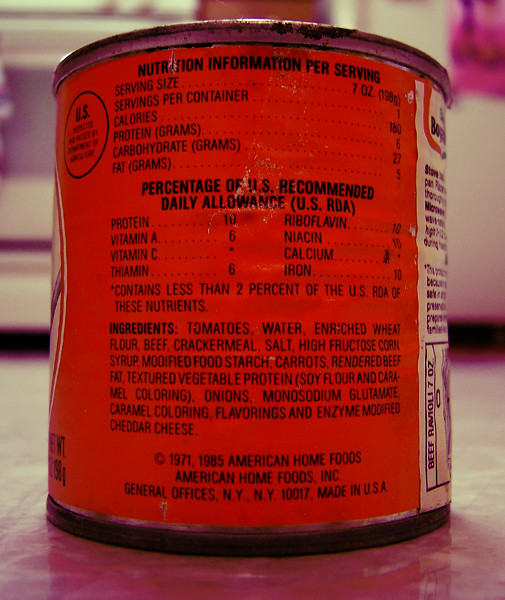This photograph captures a vintage can of what appears to be a tomato-based product, possibly something along the lines of Chef Boyardee. The can is noticeably old, with a copyright date listed as 1971 and 1985 by American Home Foods. The label features the first few visible letters of a logo, "B-O-Y," hinting at the recognizable Chef Boyardee brand.

The can is characterized by its notable rustiness at the top, emphasizing its age. It showcases a red and white label that wraps around the can. The visible back portion of the label details nutritional information per serving, followed by the percentages of recommended daily allowances of vitamins. Below the nutritional facts, a list of ingredients is displayed, with the copyright information situated at the bottom. All text on the label appears to be printed in black.

The image suggests a kitchen setting, as evidenced by the bottom half of a stove or oven visible behind the can. To the right, the lower part of a refrigerator can also be seen, grounding the scene in a domestic environment. The can itself is slightly tilted, curving off to the right side, accentuating its rounded shape and further revealing parts of the white segment of the logo.